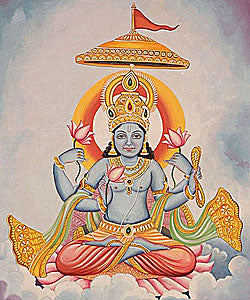An intricately detailed illustration portrays a Hindu deity seated gracefully on a fluffy cloud. The deity's legs are crossed in a meditative posture. She is dressed in vibrant red-orange pants and is bare-chested, adorned with several gold necklaces that accentuate her serene femininity. The deity's attire is complemented by a gold belt cinched at her waist and multiple arms adorned with ornate gold bangles that add to her divine aura. Her head is crowned with an elaborate, jewel-encrusted gold crown. She sports long, flowing black hair beneath an intricate, bowl-shaped gold headdress adorned with a prominent red flag.

Behind her, an elaborate orange and red decal serves as a striking backdrop. In her hands, she cradles delicate red flowers, adding to her ethereal presence. A luxurious green and gold scarf billows behind her, enhancing the sense of movement and majesty in the image. The background is textured with expressive gray and white brushstrokes, providing a subtle yet dynamic contrast to the vibrant hues of the deity and her regal adornments.